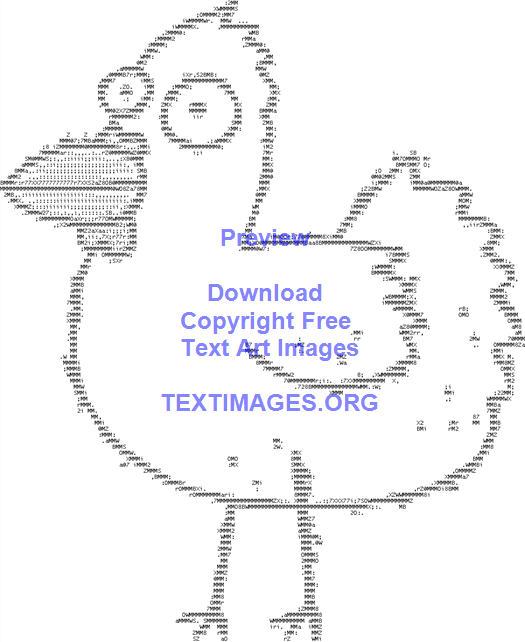This image presents a striking example of ASCII art, a form of digital illustration using text characters to create visual images, popular in the 1980s. Depicted is a whimsical cartoon chicken, featuring exaggerated, googly eyes, a comical beak, and stick-like legs and tail, all rendered in grayscale. The chicken is oriented to the left, and each aspect of the drawing is meticulously constructed from various letters, numbers, and characters, giving it a pixelated, textured appearance. Dominating the center of the artwork is a blue watermark with the text "Preview - Download copyright free text art images at textimages.org," suggesting this image serves as an advertisement. The background remains starkly white, which accentuates both the detailed ASCII artistry and the overlaying watermark.